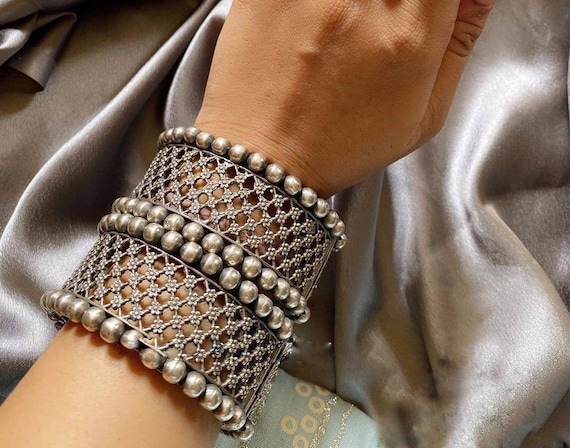In this detailed photograph, a woman's light tan, hairless left arm gracefully extends diagonally across the frame, from the bottom left to almost the top right. Her hand, hovering above a sumptuous silky silver fabric and a light blue cloth adorned with white circles and delicate silver designs, is adorned with two large, identical metallic bracelets. These bracelets, stacked one above the other just below her wrist, feature an intricate latticework structure bordered by silver or pewter beads on both edges. The lattice design includes small holes and additional beads where the patterns intersect, creating a sophisticated, elegant look. The overall scene suggests the woman might be trying on jewelry for a special occasion, set against a backdrop of luxurious, soft fabrics.